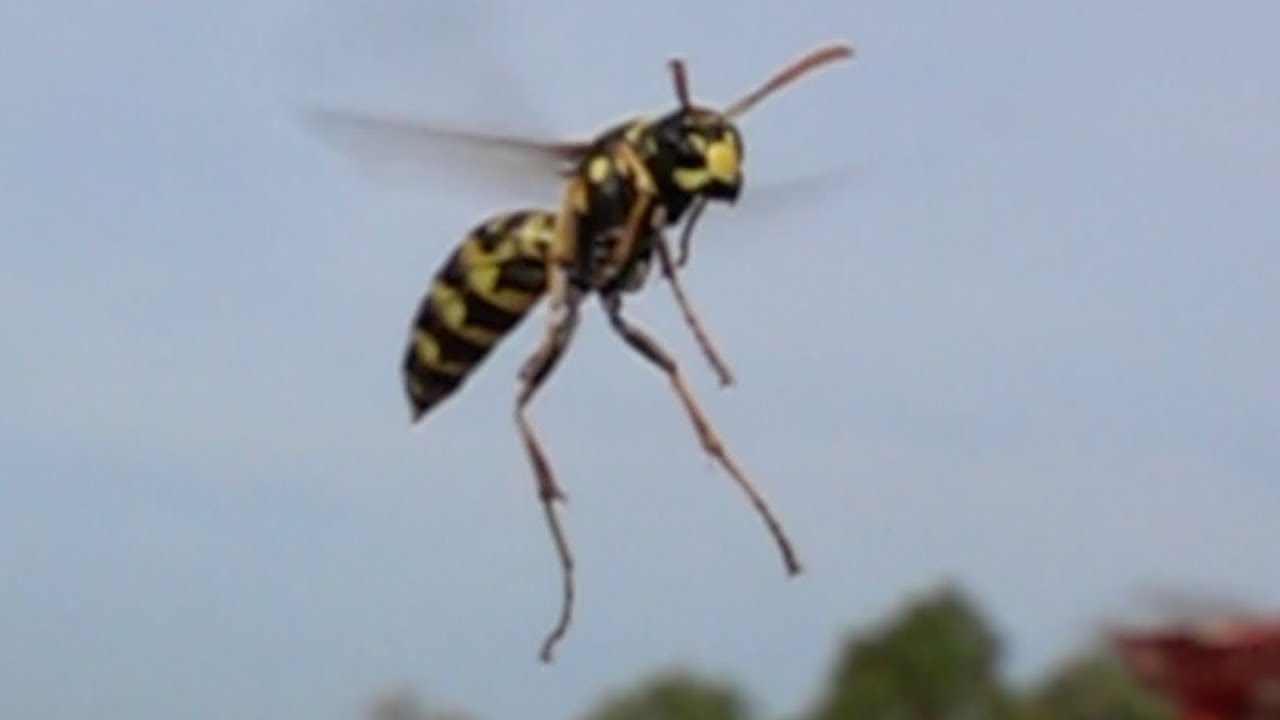This photograph captures a wasp mid-flight against a blurry backdrop of a daytime sky. The wasp, its legs trailing and wings blurred from rapid movement, stands out despite the overall lack of focus. Its striped body features bold black and yellow patterns, with additional black dots on its back and a prominent stinger. The insect's head displays distinct black eyes and yellow areas near its mouth, along with two antennae. The setting includes a light blue sky and out-of-focus tree tops at the bottom of the image, with an indistinct red object on the right side. The wasp’s elongated rear legs dangle beneath it, giving it a somewhat sluggish appearance as it flies through the air.